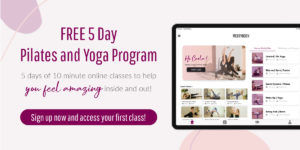In this promotional image, the design features a white background with a light pink interior encased within a light gray outlined box. On the left side, a slightly darker pink half-circle is intersected by a pinkish line. The text "Free 5-Day Pilates and Yoga Program" is prominently displayed in a darker pink font at the top. Below this, smaller gray font reads, "5 Days of 10 Minute Online Classes to Help." Further down, in a gray handwritten style, the phrase "You'll Feel Energizing" appears, followed by more gray font stating, "Inside and Out."

Toward the bottom of the image, a reddish circle contains the pink text: "Sign Up Now and Access Your First Class." An iPad outline, detailed with either gray or black lines, is situated prominently; its screen displays a white background with black text and small photographic images, though these images are not clearly visible due to their size.